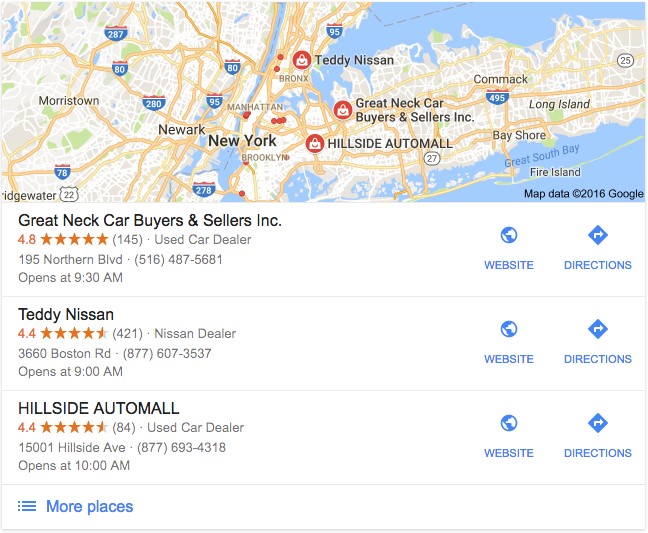The image showcases a Google Maps page focusing on several car dealerships in the New York metro area, including Brooklyn, Manhattan, The Bronx, and nearby regions like Newark and Morristown. The map is situated at the top of the page, highlighting key locations. Below the map, several listings for car dealerships are displayed prominently.

The first listing is for "Great Neck Car Buyers and Sellers," a used car dealer with a commendable 4.8-star rating from 145 reviews. It is located at 195 Northern Boulevard, and its contact number is 516-487-5681. The dealership opens at 9:30 AM and features a blue button for accessing their website along with another for obtaining directions.

Next is "Teddy Nissan," another dealership with a 4.4-star rating garnered from 421 reviews. This Nissan dealer is situated at 3660 Boston Road and can be reached at 877-607-3537. It opens its doors at 9 AM. Similar to the first listing, this one also includes clickable blue buttons for the website and directions.

Following that is "Hillside Auto Mall," which is also a used car dealer with a 4.4-star rating based on 84 reviews. The address for Hillside Auto Mall is 1501 Hillside Avenue, and their phone number is 877-693-4318. This dealership opens at 10 AM and includes navigation options to access their website and directions.

Additionally, there is a "More places" button on the webpage, suggesting that there are further listings available beyond these initial results.